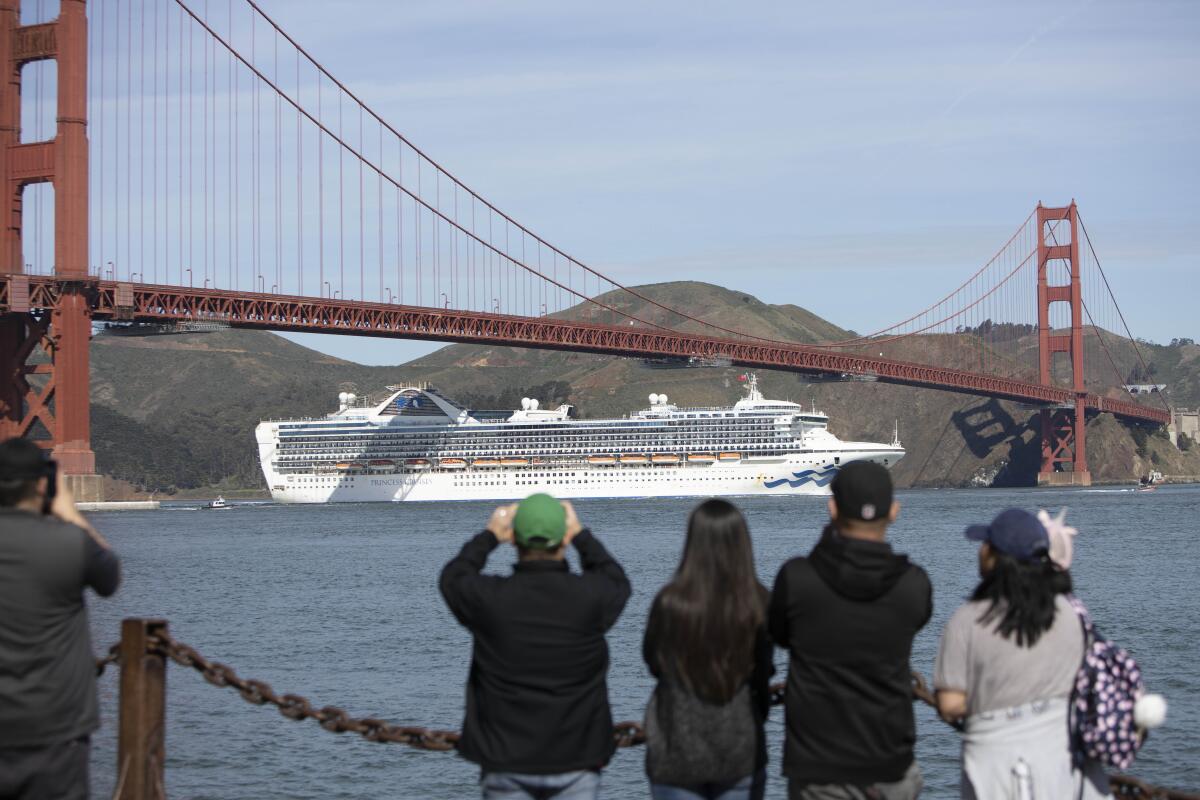The photorealistic image depicts the iconic Golden Gate Bridge in the top half, stretching majestically across a vivid blue sky accentuated with subtle, streaky clouds. Dominating the center of the scene, a massive white cruise ship, adorned with a blue ribbon-like logo on its bow and yellow lifeboats along its sides, gracefully passes underneath the bridge, appearing to nearly touch its underside. The backdrop reveals gently rolling hills, enhancing the natural beauty of the setting. In the foreground, five individuals stand separated by a chain-link guardrail, capturing the moment with their cameras. Four of the people, dressed mostly in dark clothing, are congregated towards the right, while one person is partially visible on the left. The person on the far right stands out, wearing gray clothing and holding a vibrant purple backpack. Together, these elements create a harmonious composition showcasing the juxtaposition of human scale, modern engineering, and natural landscape.